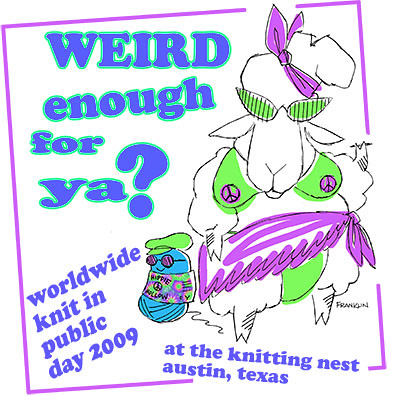This small square image with a purple border against a white background captures an eclectic scene. The border is open at the top, right, and bottom. In the upper left corner, the text "WEIRD ENOUGH FOR YA?" is prominently displayed in large blue letters, highlighted in bright green, with "WEIRD" in all caps and followed by a question mark. In the lower left corner, the text "WORLDWIDE KNIT IN PUBLIC DAY 2009" appears in a different shade of blue.

On the right side of the image, there is a whimsical depiction of a goat (some might mistake it for a sheep) adorned with green sunglasses and a purple bow on its head. The animal is humorously dressed in a green swimsuit top with outlined breasts, each marked with purple peace signs, and a purple wrap around its waist, depicted with squiggly lines. To the left of this eccentric goat, a small blue critter, possibly a spool of yarn, sports sunglasses, a green hat, and a colorful pink, green, and purple wrap. The critter carries the text "HIPPY" along with a peace sign.

At the bottom of the image, where the purple rectangular border is open, it reads "AT THE KNITTING NEST, AUSTIN, TEXAS" in blue. This bizarre yet fascinating scene ties together with a sense of quirky celebration, alluding to a unique event held in 2009.